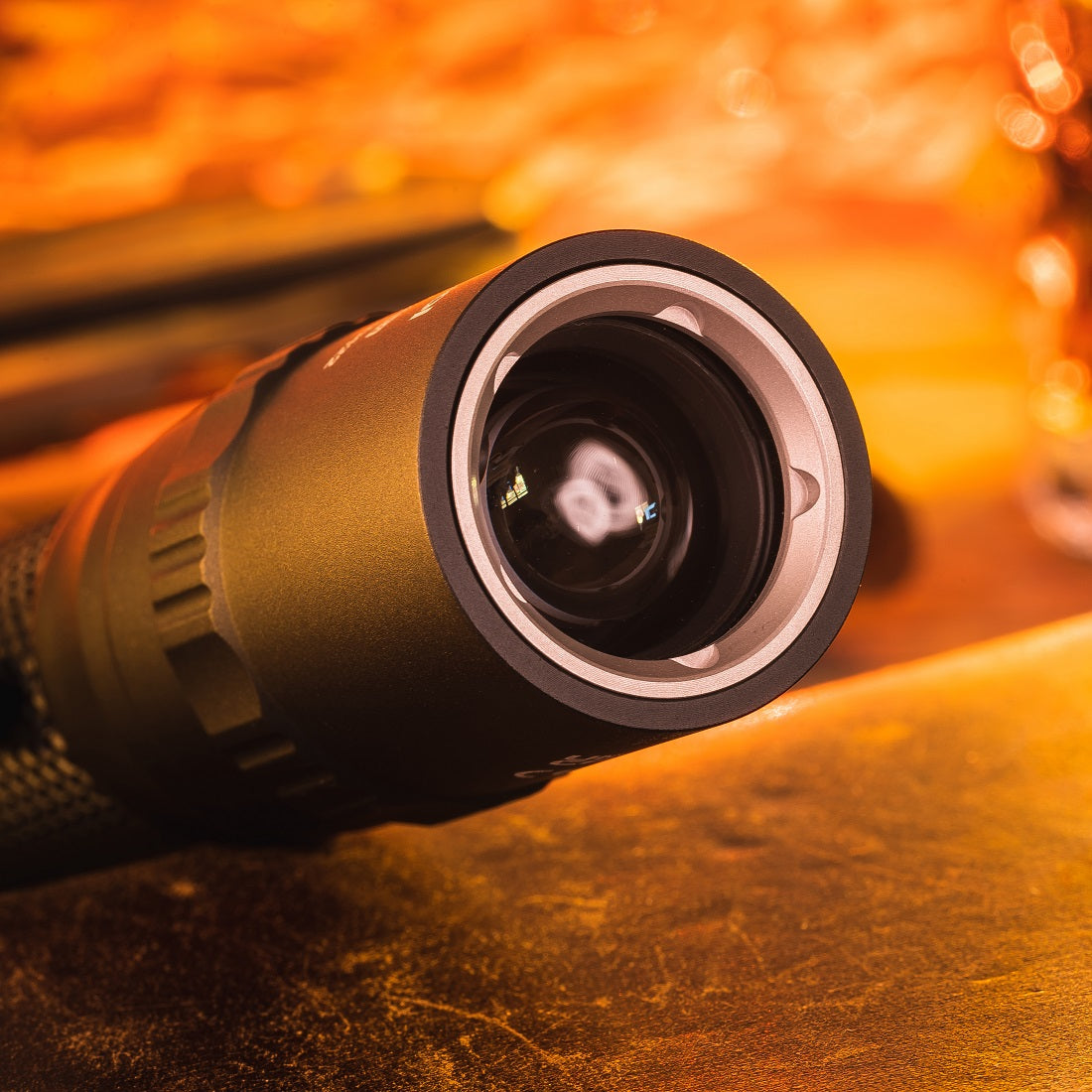This is an up-close photograph of an optical device, likely a camera or projector, centered around its black cylindrical lens. The device is positioned diagonally on a scratched, dark leather surface that occupies the bottom third of the image and is illuminated with an orange hue. The top of the frame features a blurred orange light, adding a dramatic effect to the composition. Prominent in the foreground, inset within the main black cylinder, is a silver disc encasing another black cylinder, leading down to a central glassy orb reflecting two white concentric lights. To the left of the main cylinder, there's a ridged black section and another smaller black cylinder, extending towards a slightly blurred dark gray ridged surface. The device features multiple areas where adjustments can be made, including twisting knobs situated around the textured, gear-like surfaces.